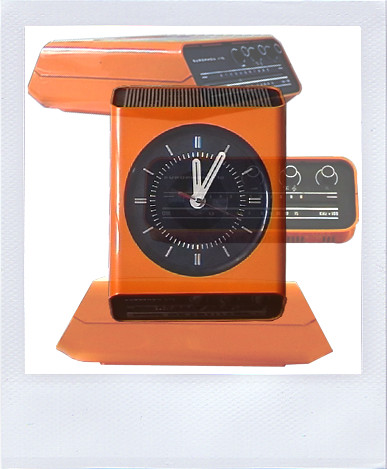This image features an orange, square-shaped, plastic desktop clock with a semi-hollow interior on a white background. The clock sits on an orange base and has a distinctive black clock face with white details, showing the time as either 12:10 or 12:05, with Roman numerals and small dots marking the seconds. The top of the device appears open with slats running across it, suggesting the capability to pour something through it. Additionally, there's a console behind or above the clock with black knobs and a black front face, possibly part of the device, adding to its layered appearance. This console looks like it could function as a radio. The entire setup gives a sense of multiple exposures, highlighting different angles and parts of the clock and its components.